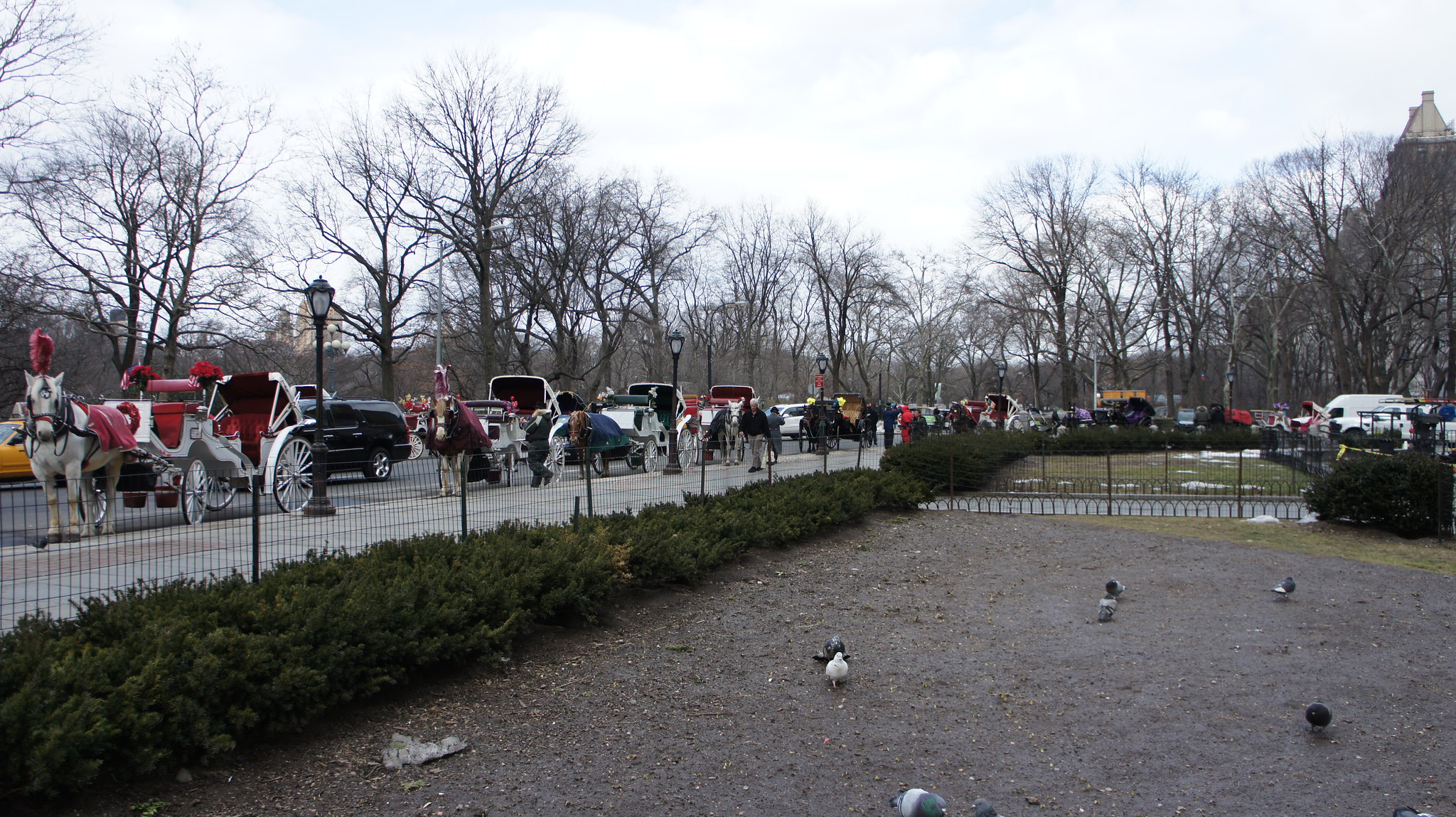This photograph captures a bustling city street, possibly in an overcast London during autumn or winter, characterized by leafless trees and grey skies. The left side of the image showcases a road with both moving traffic and several grand, ornate horse-drawn carriages. These carriages, some empty and others with dual seating areas, are helmed by impressively large horses adorned in decorative armor featuring mohawk-style helmets. Alongside the roadway, various pedestrians traverse the sidewalk past elegantly designed street lamps. On the right side of the image, a black wrought-iron fence encloses a park area where pigeons peck at the mud-covered, grassless ground. The background is dotted with indistinct buildings, and the scene’s color palette includes hues of yellow, black, red, green, and white, heightening the atmospheric ambiance of this urban locale.